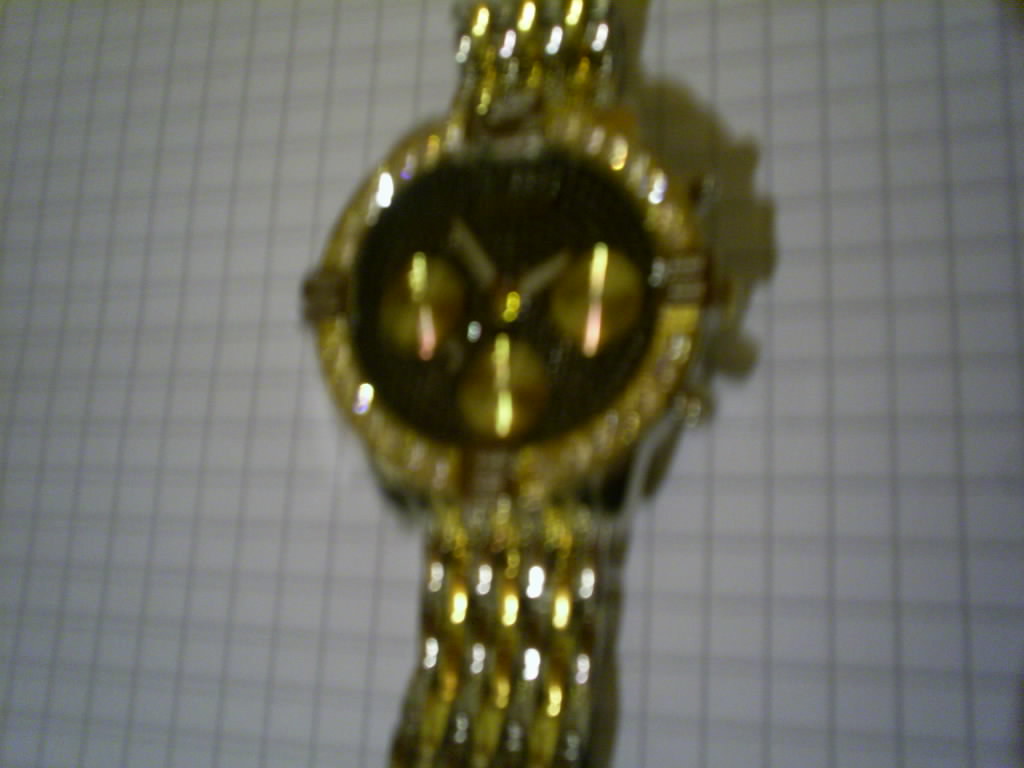This image captures a blurred photograph of a shiny, reflective watch, predominantly gold with elements of silver. The watch features a black face adorned with three gold circles that encase hints of red. The face is surrounded by white diamonds and has two golden hands marking the time, which appears to be around 2:50. The outer frame of the watch is gold, also encrusted with diamonds. The band of the watch is a sophisticated blend of gold and silver, arranged in a braided pattern. The watch is laying on a white graph paper with dark lines, casting a subtle shadow towards the right, suggesting the light source is coming from the left. The overall image is somewhat blurry and seems to have been taken with a personal camera, giving it an intimate and candid feel.